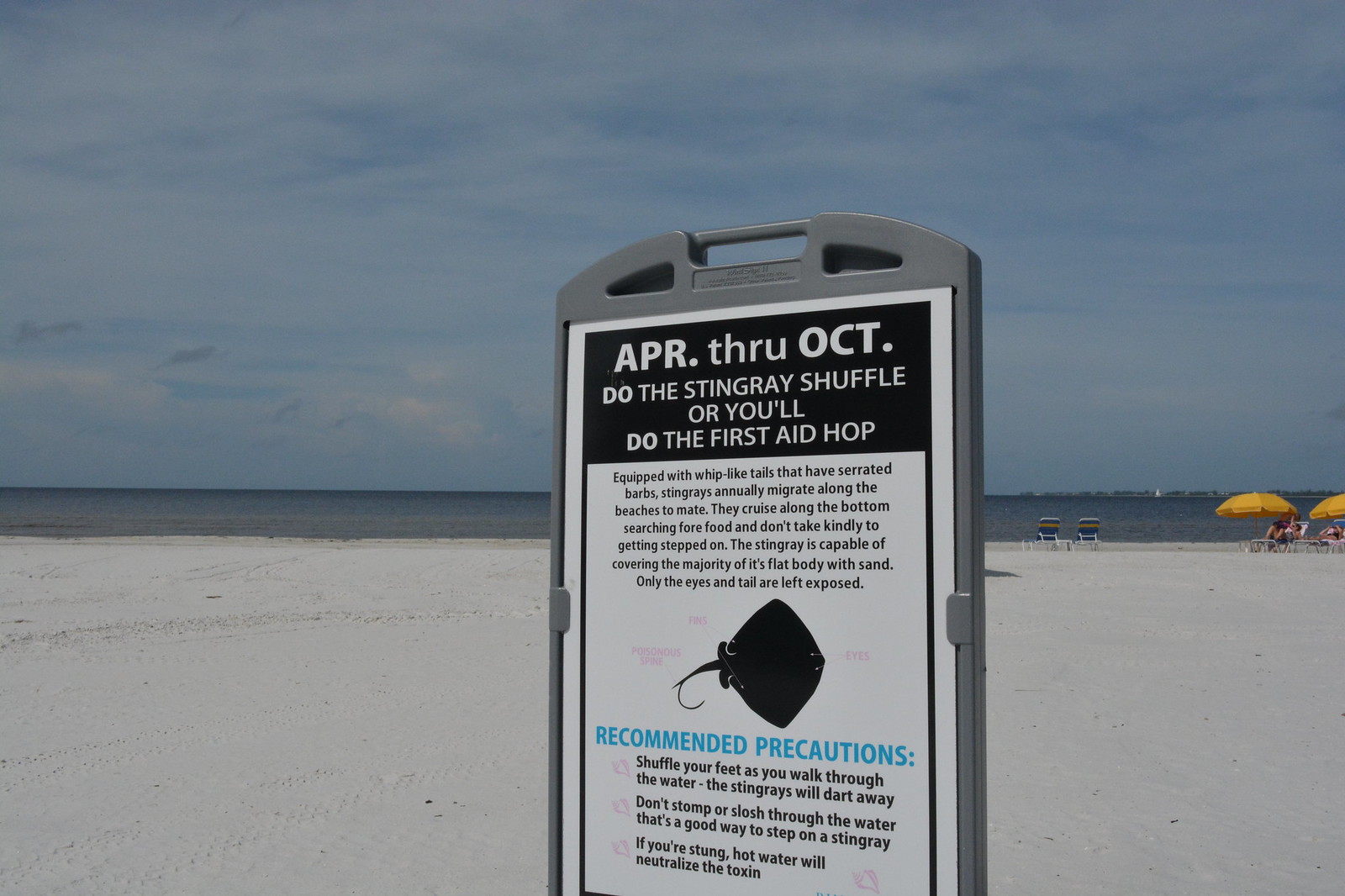On a serene beach with white sand stretching to a deep blue ocean under a partly cloudy sky, a prominent gray sign with a white center stands as the focal point of the image. Positioned centrally in the photograph, the sign relays an important safety message in black and white text. The top of the sign reads, "APR through OCT, do the stingray shuffle or you'll do the first aid hop," warning visitors about the stingray season from April to October. It provides detailed instructions on avoiding stings by shuffling feet through the water instead of stomping, as stingrays, with their whip-like tails and serrated barbs, migrate annually and can be hidden beneath the sand. Precautionary measures and first aid tips, such as using hot water to neutralize the toxin, are also listed. To the right of the sign, two yellow umbrellas provide shade for a few beachgoers sitting in chairs, emphasizing the peacefulness of the relatively empty beach scene. To the left, two empty chairs overlook the tranquil waters, enhancing the overall calmness of this coastal setting.